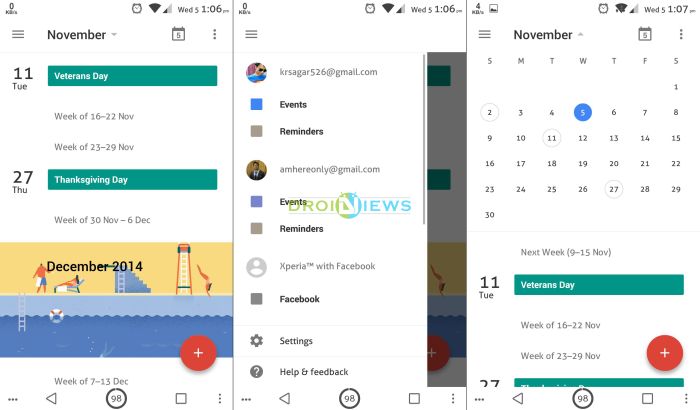This image comprises three side-by-side screenshots of a cell phone interface. 

- **Left Screenshot:** Displays a partial calendar view for November, highlighting significant dates such as Veterans Day on the 11th and Thanksgiving Day on the 27th, but no personal events are recorded. Only notable public holidays are visible in this streamlined calendar summary. 

- **Middle Screenshot:** Features a menu screen presenting various sections such as events and reminders tied to different email accounts associated with the device. This menu serves as an aggregation point for managing and integrating tasks into the calendar. 

- **Right Screenshot:** Showcases a detailed, full-page calendar for November, outlining all days of the month. Below the monthly view, specific details for each day are noted, with Veterans Day highlighted on Tuesday, the 11th. The subsequent two weeks appear to have no listed events. 

All screenshots display the typical cell phone status icons at the top, indicating the device's Wi-Fi connection, an active alarm, and the time, which transitions from 1:06 to 1:07 PM on a Wednesday during the screenshots capture.